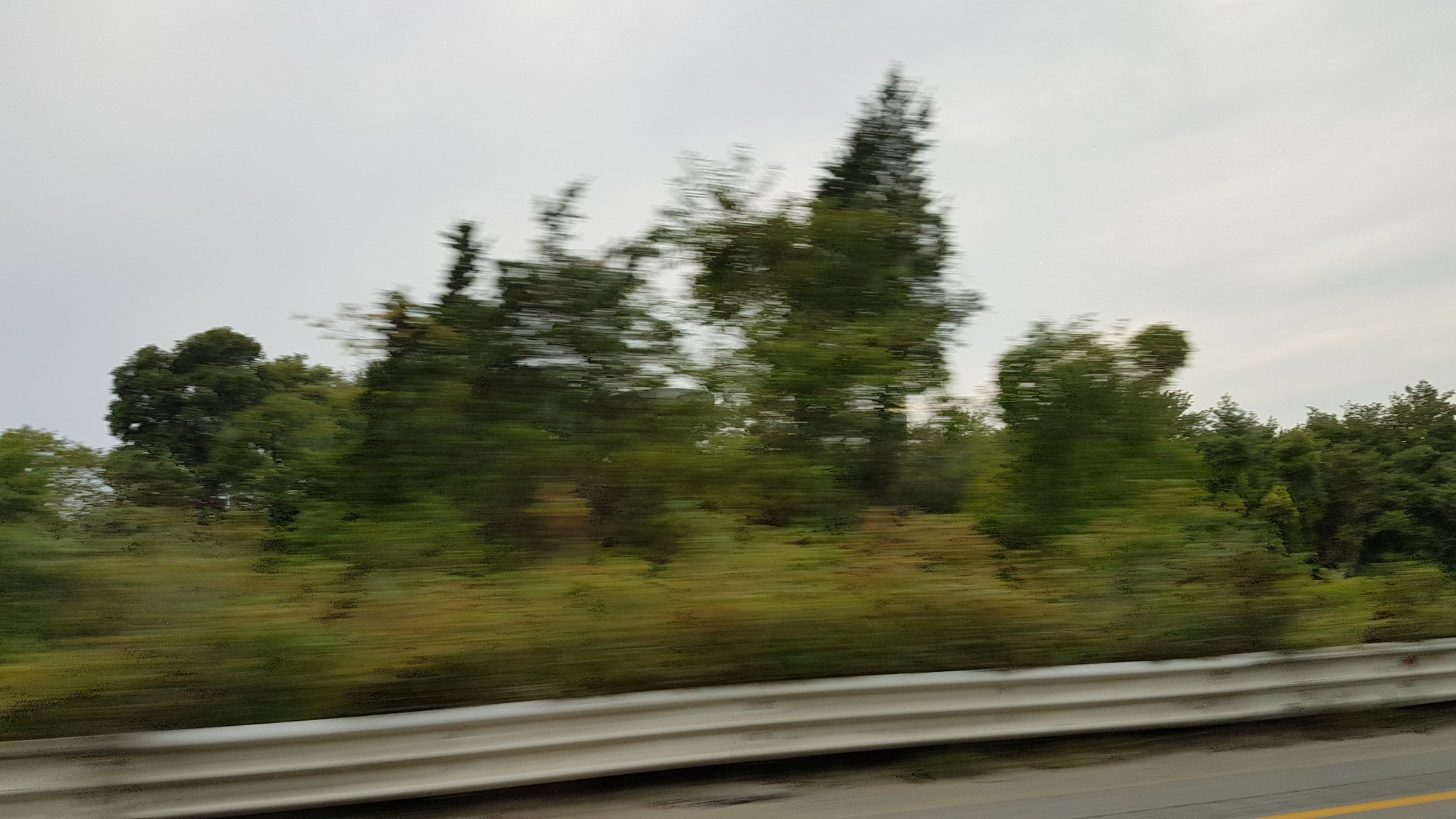This is a blurry photograph taken from a moving car, capturing the side of a road with the perspective slightly angled, indicating the road runs from right to left on a gentle slope. In the foreground, at the very bottom of the image, you can see a small yellow stripe on the pavement. Just above this, the characteristic metal corrugated guardrail common along American highways is visible. Beyond the guardrail, there is a mix of greenery including bushes, hedges, and patches of grass. The backdrop is filled with a variety of trees, including tall pines and more rounded trees, all in different shades of green. The sky above is overcast with a bright but gray hue, containing some barely discernible ruffled clouds. There is no direct sunlight casting shadows on the scene, adding to the soft, diffused light effect.